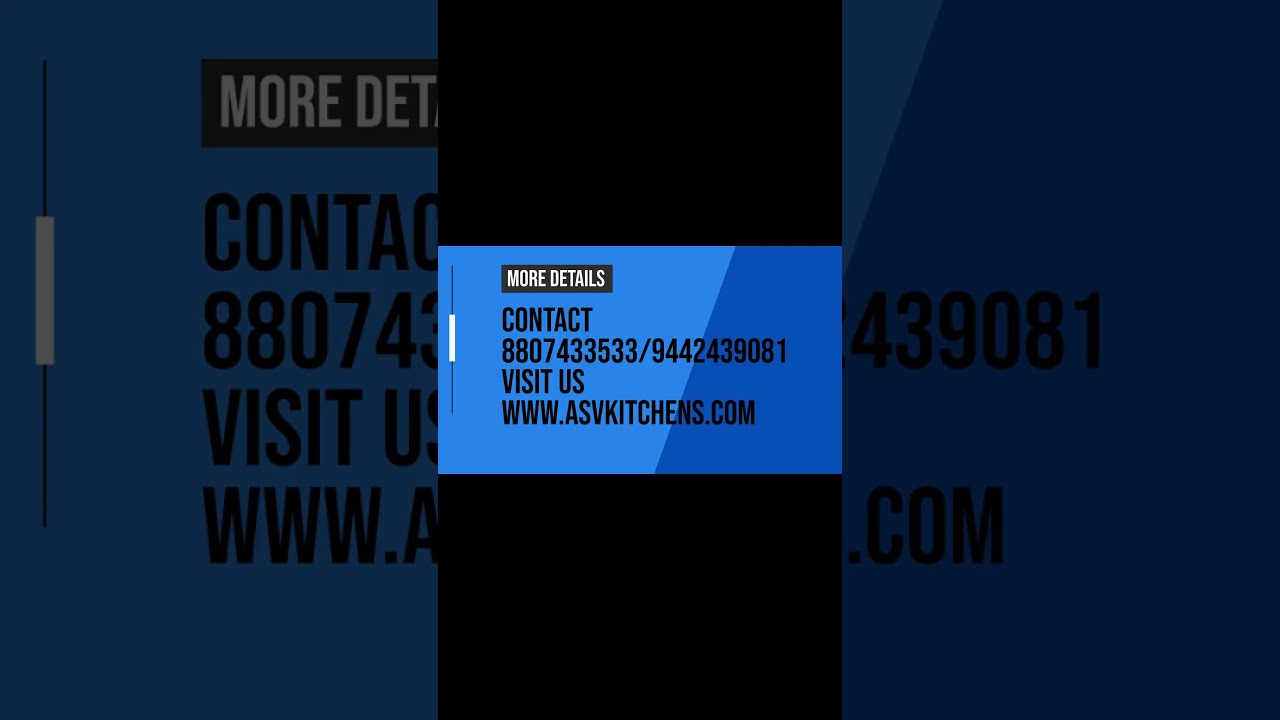This horizontal rectangular image features a dark blue background with faded, zoomed-in portions of the central content, creating a layered effect. The centerpiece is a prominently displayed vertical rectangle designed to resemble a business card. It has solid black borders on the top and bottom edges, while the center background is divided by an oblique line into two shades of blue—light blue on the left and dark blue on the right. Within this central rectangle, the text, all in capital letters, reads: "MORE DETAILS" in white, followed by "CONTACT 8807-433-533/944-243-9081" and "VISIT US WWW.ASVKITCHENS.COM" in black. The text is left-aligned, enhancing the information's readability against the blue backdrop.